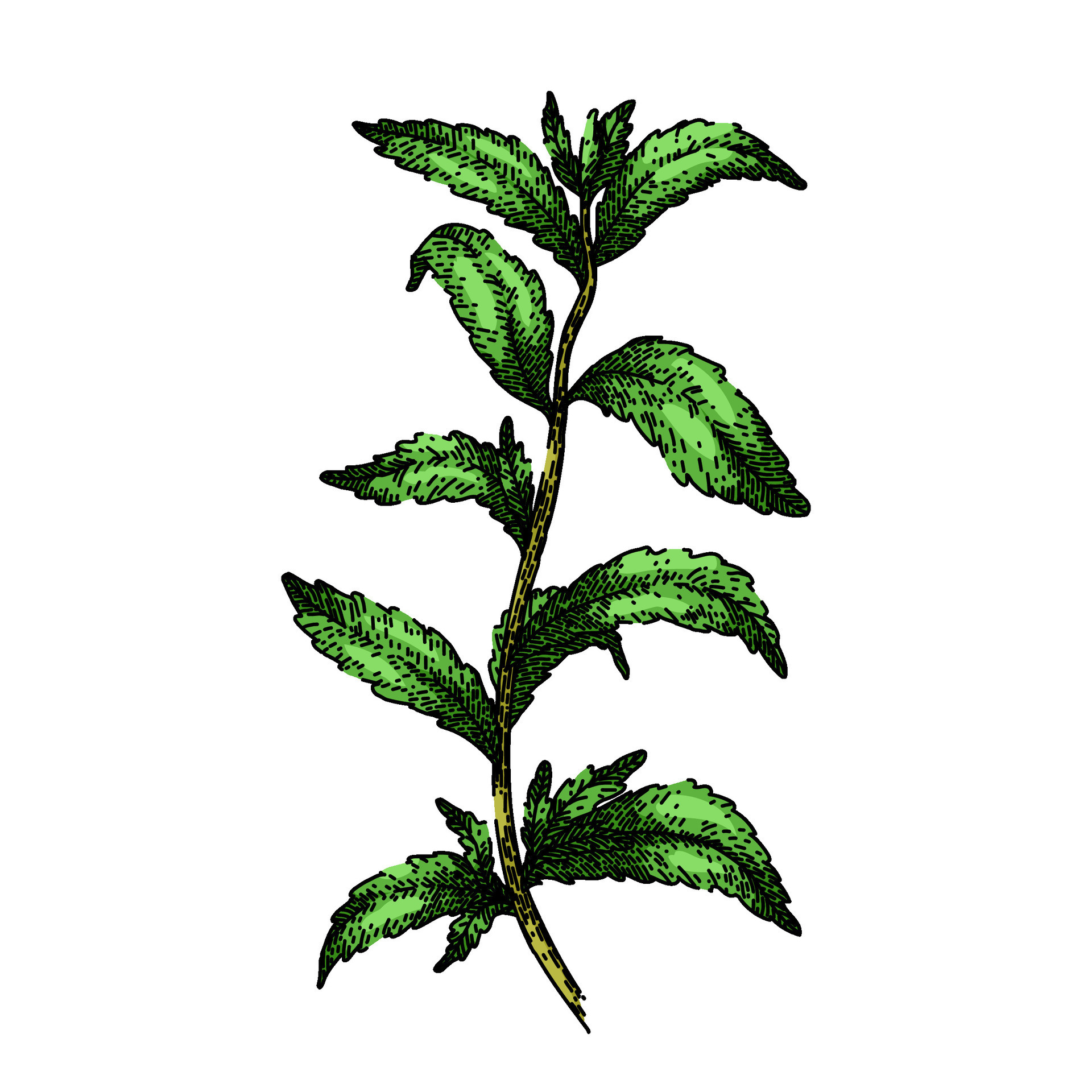This digital image depicts a stylized, pixelated drawing of a tall plant with a light olive green stem, accented with black lines indicating shadow and texture. The stem is slightly curved and runs from the base to nearly the top of the image, which features contrasting green leaves. The leaves are predominantly medium green, with darker tones at the edges and lighter green highlights in the center. Starting with a small cluster of three leaves at the top, the plant features nine leaves positioned along the length of the stem, morphologically diverse with some long and floppy, exhibiting a mix of shades from light to dark green. The bottom section of the plant is accentuated by two sets of leaves, each larger leaf accompanied by two smaller ones, arranged three on the right and three on the left. The image has a stark white background, ensuring that there are no distractions from the detailed plant rendering. This artistic representation captures the essence and structure of the plant in a unique, almost abstract style.